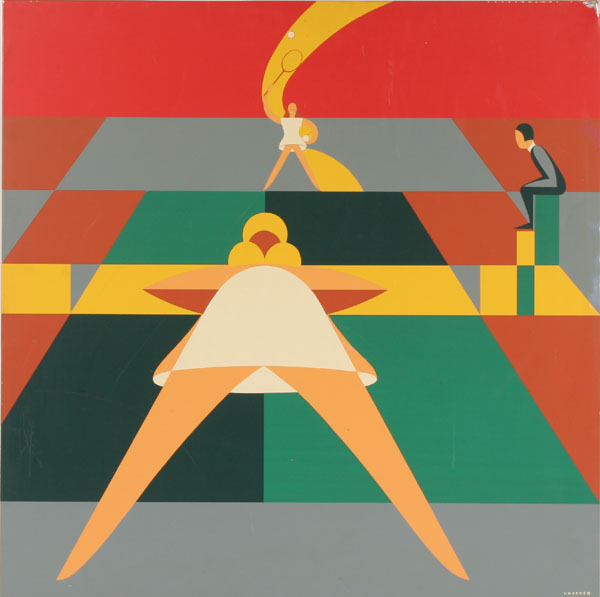The image is a highly detailed and modernistic art project depicting a tennis game in progress using a cubist style with digitally created shapes. The scene features two women dressed in tennis whites. The woman in the foreground, possibly with blonde hair or a yellow hat, is bent over, ready to receive a serve, her posture accentuating the tension of the moment. Her legs, depicted as beige triangles, complement her curved skirt. On the other side of the net, constructed from blocks of orange, green, and blue squares, the second woman is poised to serve, holding a white tennis ball in her hand and her racket above her head. Behind the serving player is a yellow band, adding to the dynamic composition. At the center, seated on a green rectangle, is a faceless judge, attentively observing the match. The background is a mosaic of colorful squares, including shades of red, yellow, white, gray, orange, and green. The entire scene, framed by a red border at the top, captures the essence of a competitive tennis match frozen in motion, all depicted through a meticulous assemblage of various shapes and colors.